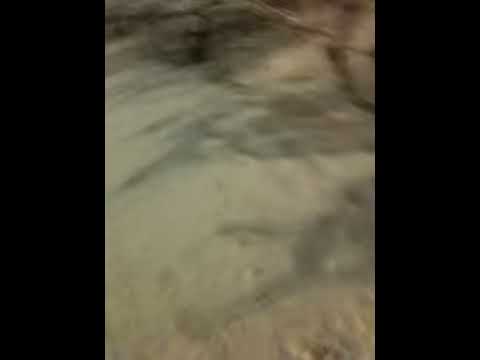This image is a blurry and pixelated photograph with a horizontally rectangular orientation, measuring about four inches wide and three inches tall. Dominating the left and right sides are thick black borders, each roughly three quarters of an inch wide. In the central section, we appear to be looking at an outdoor scene during the daytime. The photograph primarily features a tan to brown-colored ground with some variations in texture and color. Towards the lower right corner, the ground appears hard-packed with a brown hue, shifting to a greener tone as it extends upward and leftward. Shadows are present but blend indistinctly with the ground, making it difficult to identify their sources. The upper portion of the image suggests vague outlines that could be interpreted as sticks, a makeshift fence, or possibly large stones. Overall, the extreme blurriness and lack of clear definition make it challenging to ascertain precise details or the exact nature of the objects depicted.